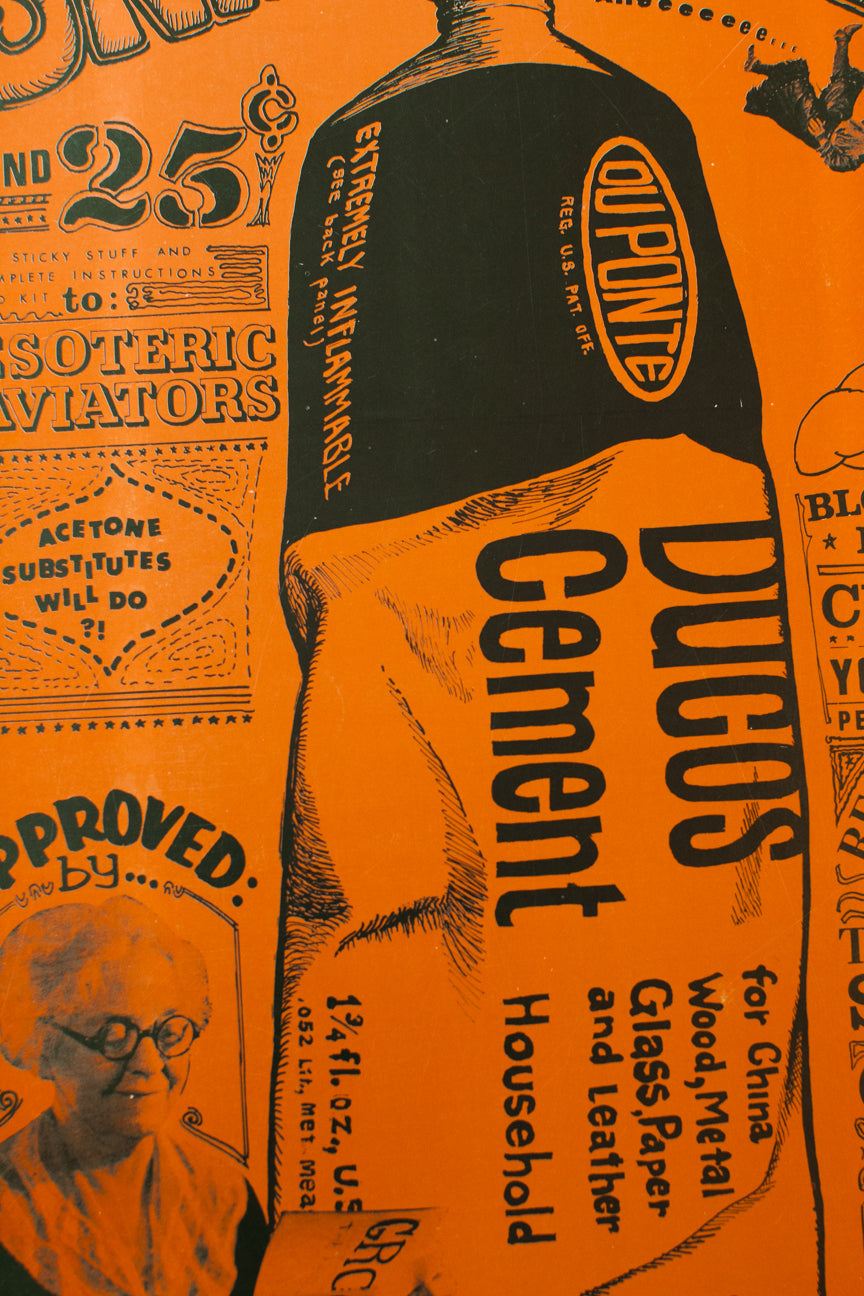This orange poster prominently showcases an illustration of a DuPont product, specifically a tube of DuCoast cement. The tube, appearing similar to a toothpaste tube, is mostly black with an orange oval at the top featuring the DuPont logo. The label on the tube reads "Extremely Flammable" and details its use for various materials: China, wood, metal, glass, paper, and leather. The entire poster, rendered in tones of orange and black, is part of a series of advertisements and includes a somewhat cut-off section about aviators on the left. In the lower left corner, there is a photograph or drawing of an elderly woman with round bifocals reading, accompanied by the text "Approved By." This juxtaposition suggests a seal of approval, adding a human element to the advertisement. The right side of the poster is partially cut off, obscuring another object next to the tube of cement.